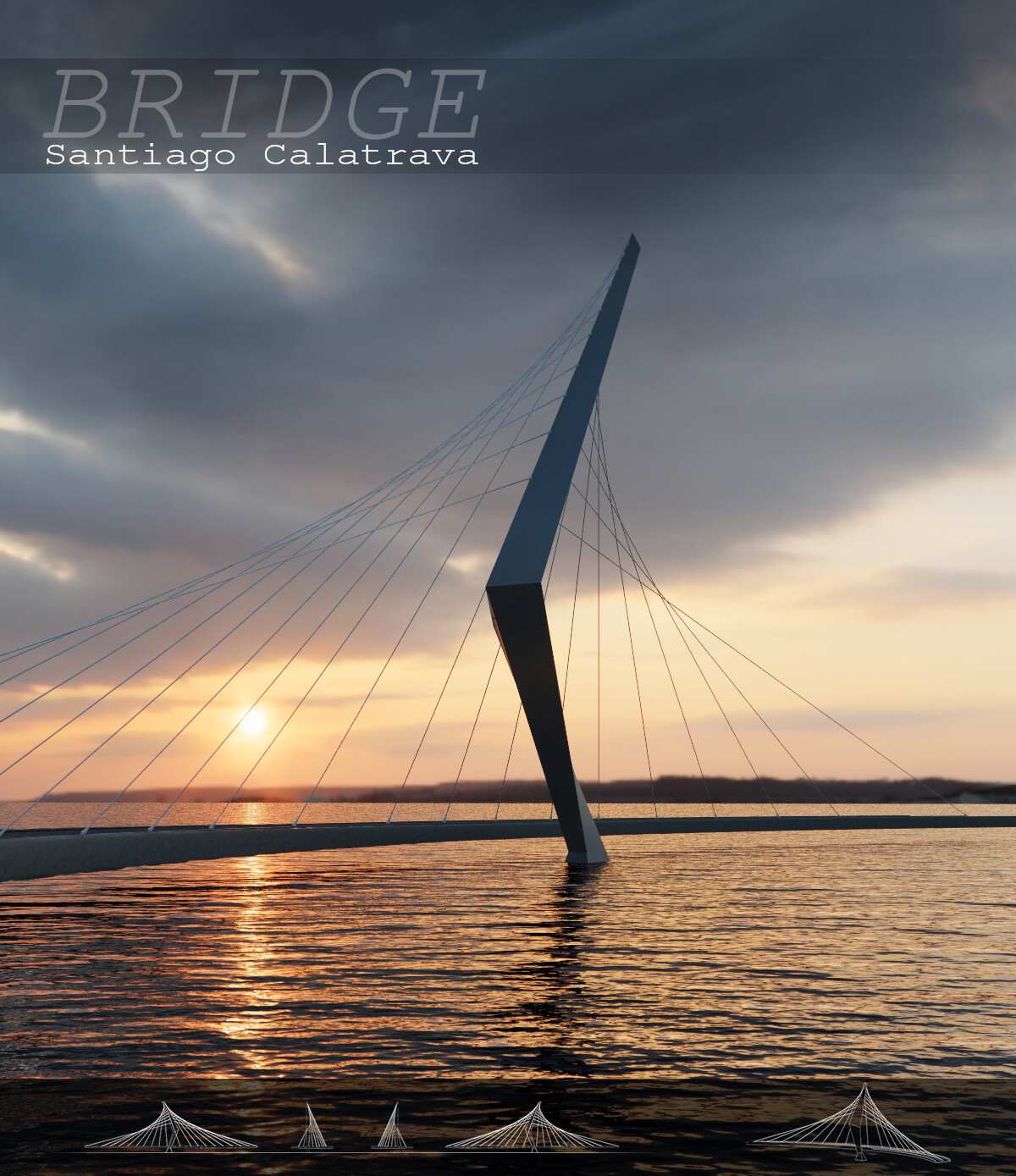This is a striking professional photograph capturing a modern suspension bridge designed by Santiago Calatrava. The bridge spans across a tranquil lake or ocean, with its sleek, angled support beam and an intricate network of stretched supporting cables creating an elegant centerpiece. The sun, either setting or rising, casts a warm glow on the scene from the horizon, illuminating the dark clouds in the sky with vibrant hues of orange. In the top left corner of the image, the word "BRIDGE" is prominently displayed in all caps, with "Santiago Calatrava" written beneath it in smaller letters. The lower half of the image reveals the calm surface of the water, which mirrors the bridge's structure. At the very bottom, a thin, semi-opaque black border showcases white illustrations, possibly technical blueprints, of the bridge from various angles. This meticulously detailed composition highlights the architectural prowess and serene beauty of the scene.